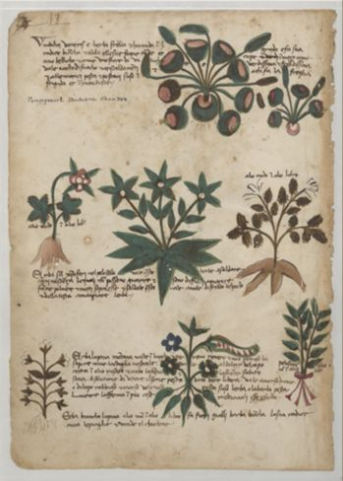The image features a vertically aligned rectangular sheet of old, off-white or manila-colored paper, bordered on all sides and appearing slightly worn with a ripped edge on the right and a partially cut-off upper left corner. This sheet seems to be a cutout page from an old book, containing various illustrations and text that is written in cursive and brown but too small and blurred to read. At the top center, there are two plant-like images; the left one depicts green buds with hints of red or pink centers and is slightly larger compared to the similar plant to its right. Below these, the middle section showcases an intricate pattern composed of star-shaped green leaves leading into a larger star-shaped flower with a yellowish base on the left and more star-like flower patterns on the right in a light brownish-pink hue. Further down, three more plant illustrations are aligned horizontally, featuring diverse leaf shapes and flower colors— the left plant has a red flower with green leaves, the middle is all green with three flowers, and the right one is primarily brown. At the bottom, another row of three plants is displayed: one brown, one green and blue, and one green with a touch of red. Throughout, there is text interspersed among the images, with paragraphs located at the top, middle, and bottom, as well as some writing in the middle right section, all of which remain indecipherable due to their small size and unfocused nature.